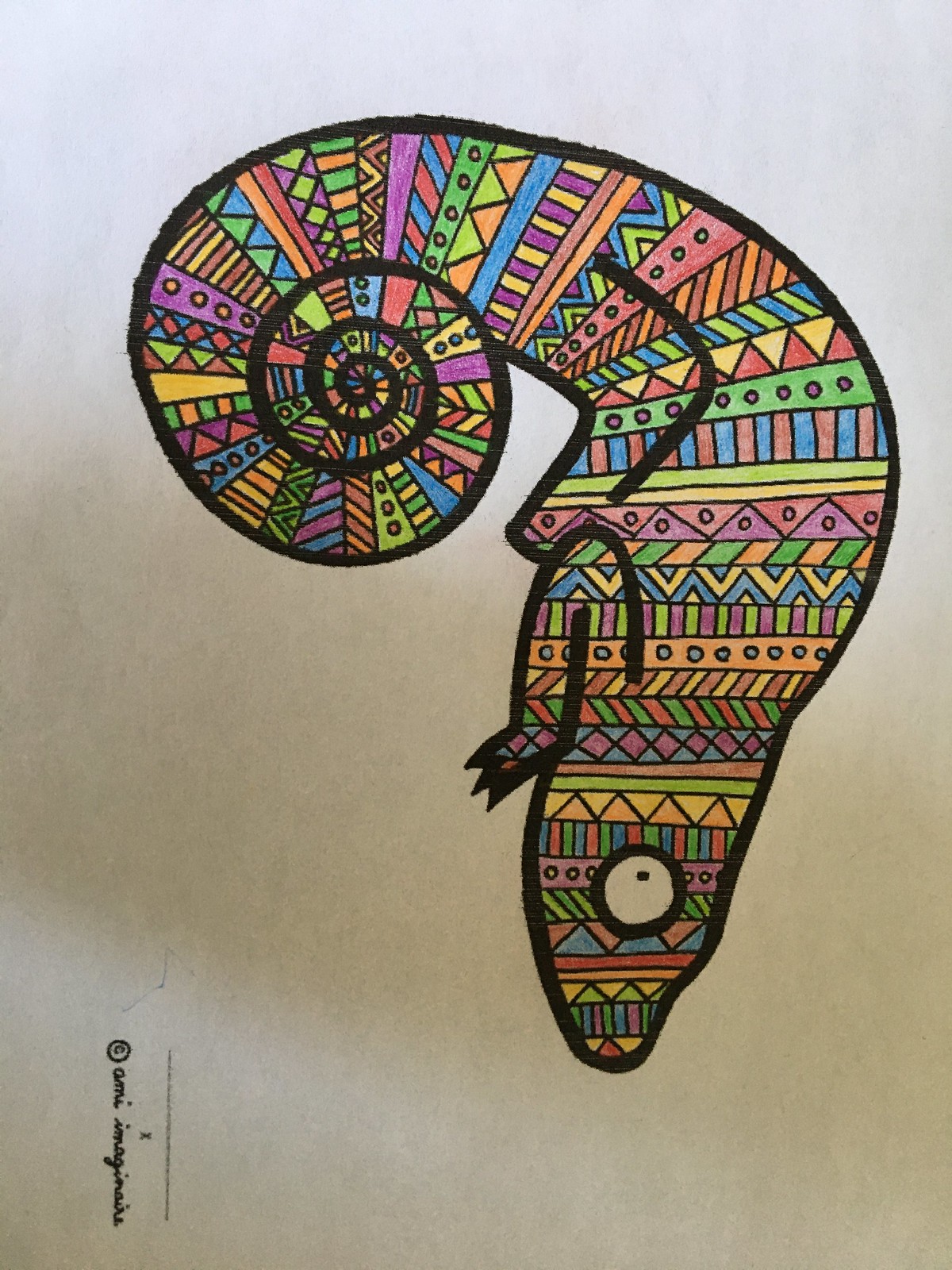This vibrant color photograph captures a meticulously detailed drawing on a whitish piece of paper. The photograph, taken from a top-down perspective, reveals a subtle shadow cast in the center, suggesting a light source from above. The paper exhibits a gradient effect, with the top portion appearing white, transitioning to a brownish hue in the middle, and lightening slightly towards the bottom. 

At the bottom edge of the drawing, oriented vertically but requiring a 90-degree rotation to the right for better legibility, there is a signature and a small copyright symbol inked in black, though the signature text is too tiny to decipher clearly.

The drawing itself features what seems to be a fantastical creature resembling a lizard, amphibian, or perhaps even a snake. The creature has a pointed head and a tail intricately curled into a spiral shape reminiscent of a snail's shell. Its body is adorned with elaborate, Aztec-inspired stripes that are divided into various geometric patterns, including diamonds, triangles, and spots. The patterns are rendered in vibrant, multi-colored hues including green, blue, yellow, red, pink, and purple, bringing a lively and captivating complexity to the creature's form.